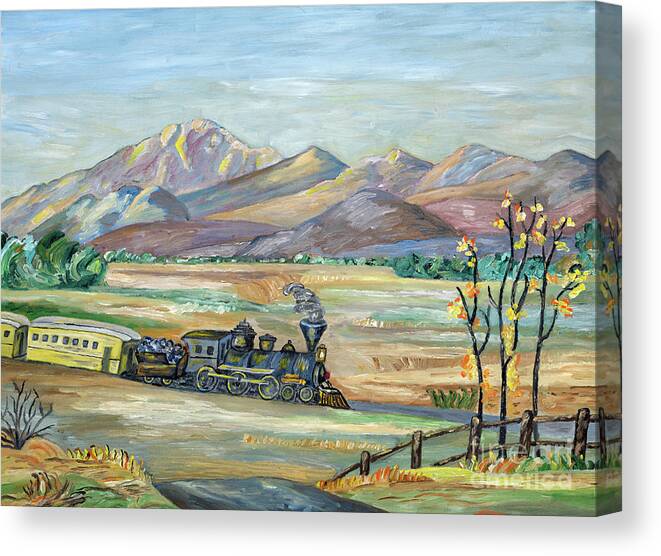The image depicts a vibrant painting, potentially crafted by an amateur artist, featuring a dynamic outdoor scene often seen in museums or personal collections. Dominating the central foreground is a black steam train, characterized by a prominent smokestack emitting puffs of smoke, chugging along a track from the left towards the right. Trailing the locomotive are four cars, with the closest and subsequent ones painted in shades of yellow and capped with white tops and windows.

Behind the train, the terrain unfolds into rolling fields adorned with various hues of greenery and bluish vegetation, accentuated by additional elements like a roadway and a quaint white picket fence encircling a tree in the lower right corner. The background elevates into an imposing mountain range, with the tallest peak situated on the left, showcasing a cascade of colors from purples and blues to oranges and reds. Above the mountains, the sky transitions from a serene blue to areas tinged with gray, suggesting a blend of clear and cloudy weather conditions. There are also subtle yellowish touches on the lower slopes of the mountains and around the scene, suggesting sunlight hitting certain patches. The landscape and artistic style, marked by bold, varied colors and simplified forms, exude a naive, whimsical charm, reminiscent of childlike creativity.